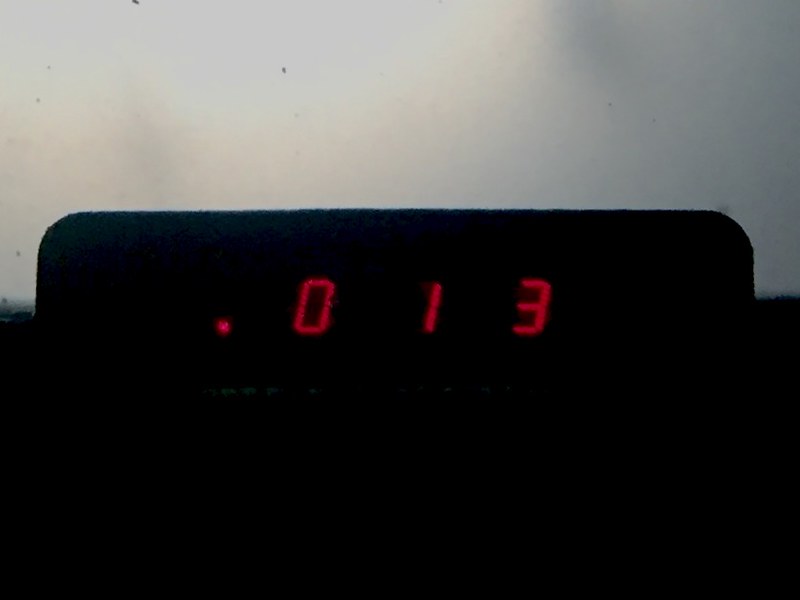A close-up image portrays an object presumed to be an alarm clock, resting on a flat surface. The object features a rectangular silhouette with curved edges, though its finer details remain obscured. The background is a soft, blurry silvery-gray, creating a subtle contrast against the object. Despite the low light conditions, three numbers are distinctly visible on the clock's display, illuminated in red LED: a solitary dot, followed by the digits '0', '1', and '3'. The red numbers stand out starkly against the otherwise indistinct features of the clock, subtly highlighting the time or another numeric display.